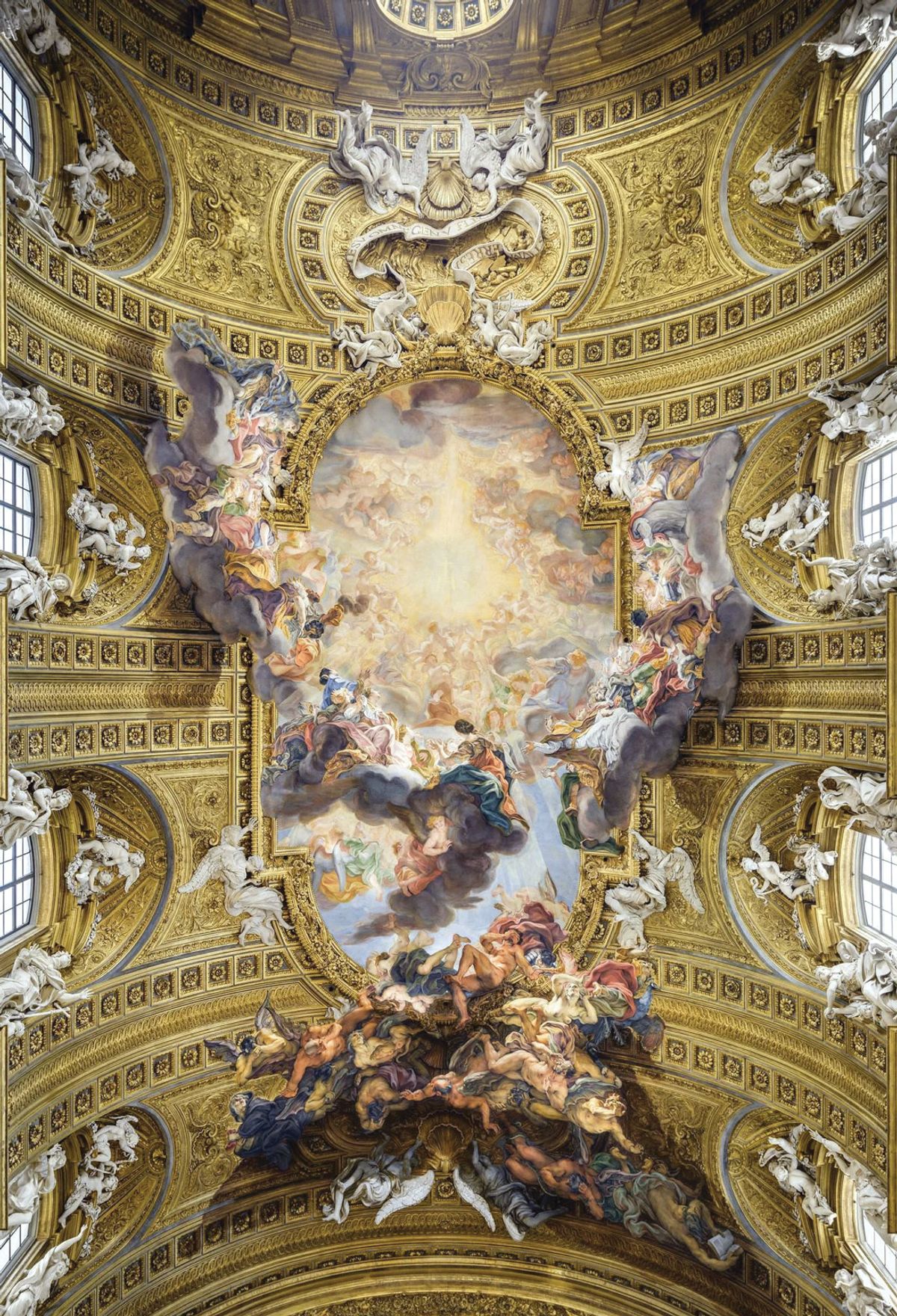The image depicts an upward view of an ornate church ceiling, possibly the Sistine Chapel. The architecture features a domed, round ceiling lavishly adorned with shiny, gold paint. Flanked by large, arched windows on the left and right, the windows are surrounded by statues of white stone angels. The center of the ceiling showcases a complex, pill-shaped mural divided into segments. The mural is filled with numerous figures, likely angels, converging towards the center, which is ablaze with a glowing yellow area, creating an impression of transportation or ascension to heaven. The intricate design of the ceiling includes tiny squares forming elaborate patterns, emphasizing the celestial theme.